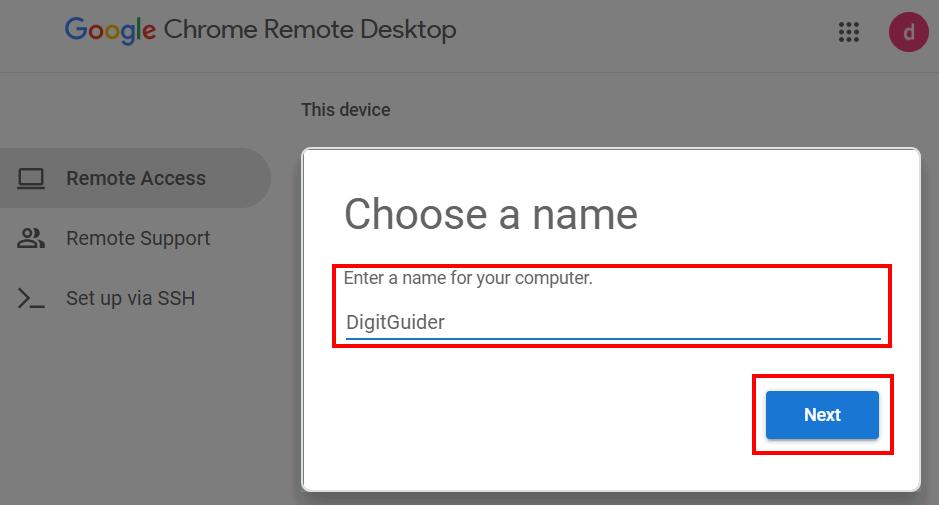On the Google Chrome Remote Desktop page, a user is signed in, indicated by their icon featuring a lowercase 'd' in the top-right corner. On the left side of the interface, there is a panel with two overlapping layers; the background layer is dimmed and grayed out, yet still shows three main sections: Remote Access, Remote Support, and Setup via SSH. The user has clicked on the Remote Access section and is currently navigating the settings. 

A dialog box has appeared, prompting the user to choose a name for their computer. The user has entered "DigitGuider" (with a capital 'G' in Guider). The name field is highlighted with red outlines, indicating that it might require additional input or corrections. Below the name field, there is a prominent "Next" button, ready to be clicked to proceed with the setup.

This process sets up Remote Access, allowing the user to control another computer from their own, or vice versa, after completing the necessary configuration steps.